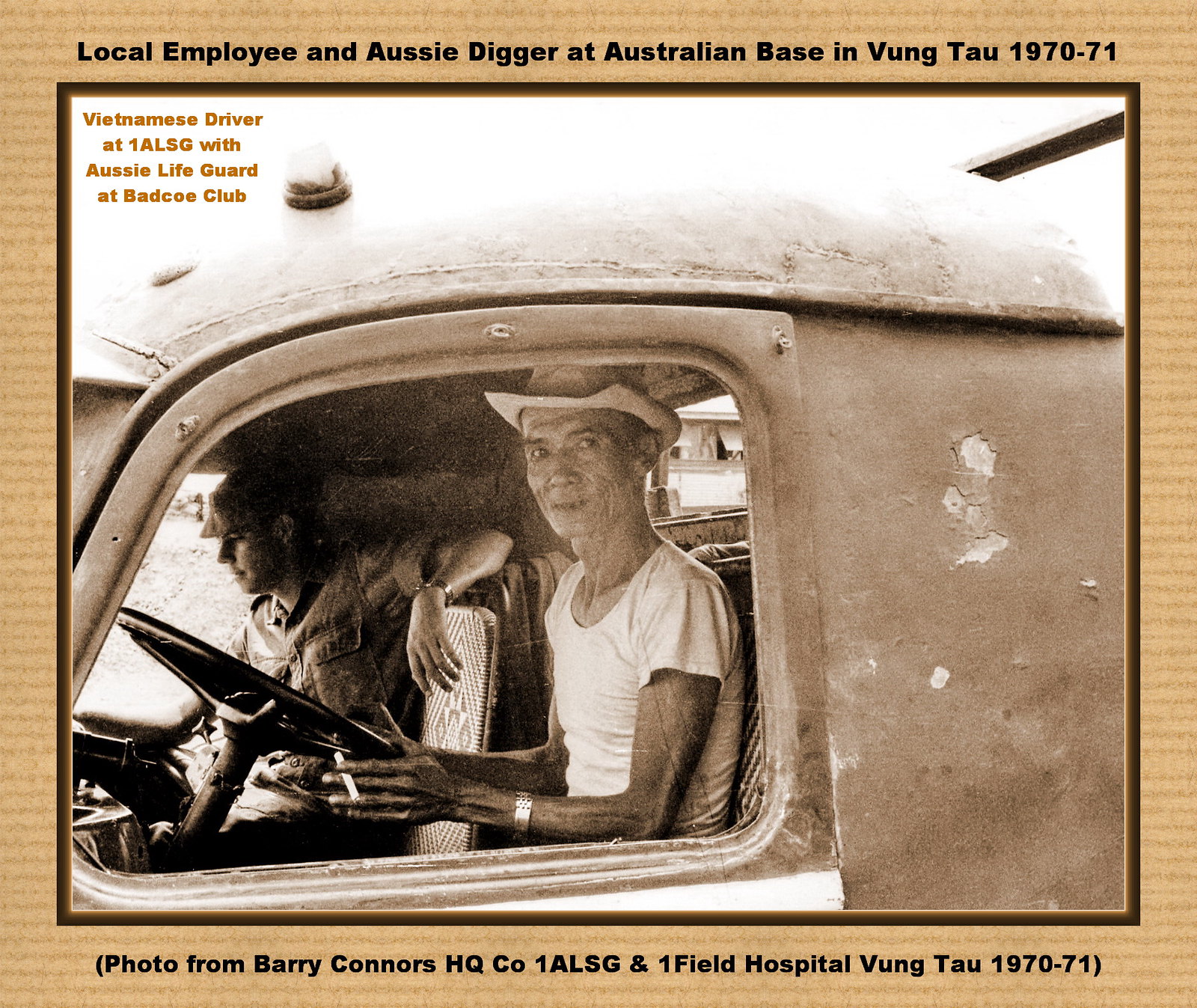The photograph, encased in a light brown, corrugated cardboard-style frame, captures a moment from 1970-71 at an Australian base in Vung Tau. Above the sepia-toned image, black text reads: "Local employee and Aussie digger at Australian base in Vung Tau 1970 to 1971." The bottom text credits it: "Photo from Barry Connors, HQ Co 1 ALSG and 1 Field Hospital Vung Tau 1970-1971." Within the frame, an older, extremely thin Vietnamese driver, clad in a white t-shirt and metal watch, holds a cigarette in his left hand while steering the old, paint-chipped vehicle. His cowboy-style hat adds to his distinct appearance. Beside him, a younger man in a t-shirt and possibly a flat cap, not looking at the camera, props his arm on the backrest, appearing neutral. The driver’s slightly malnourished look contrasts with his happy expression as he looks towards the camera. Overlaying the top left corner of the photo in brown text is a description, "Vietnamese driver at 1ALSG with Aussie lifeguard at Bag Co Club."